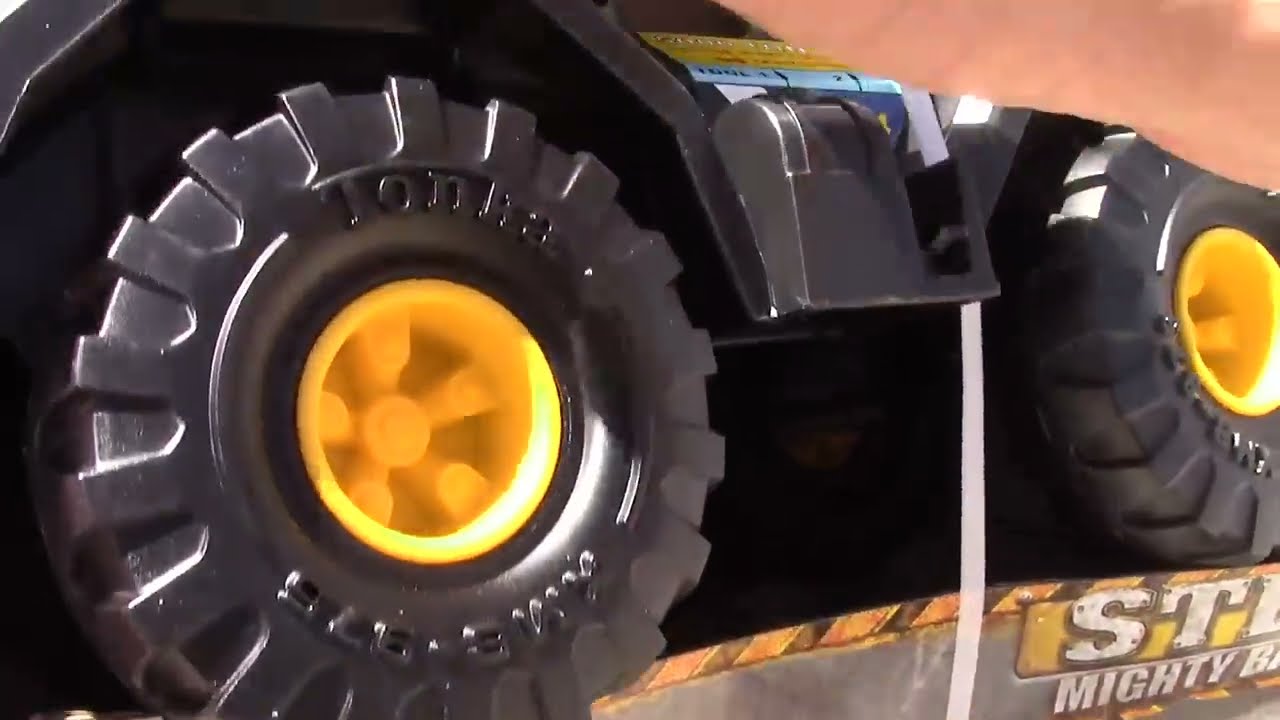The image showcases a tightly zoomed-in view primarily featuring the wheels of a Tonka toy truck, giving an extreme close-up perspective. Dominating the scene are the large, black plastic tires, each adorned with bright yellow, sunny hubcaps that lend a cheerful touch. The wheels appear hefty and durable, designed for rough play. The partially visible truck is black, possibly resembling a Jeep or a similar model, though the specific details of the vehicle are obscure. A gray bar, attached to the truck, shows the text "ST" with "MIGHTY" beneath it, partially cut off. There's also a light blue tag visible near the top portion of the image. In the setting, which seems to be indoors, possibly in a toy store, the truck is fastened to its packaging with the aid of a zip tie and a plastic strap. In the background, a tan colored backdrop is faintly discernible. Additionally, a part of a hand is seen at the upper right corner of the image, adding a sense of scale. The lower right corner reveals the edge of the cardboard box containing the toy with some partially readable text.